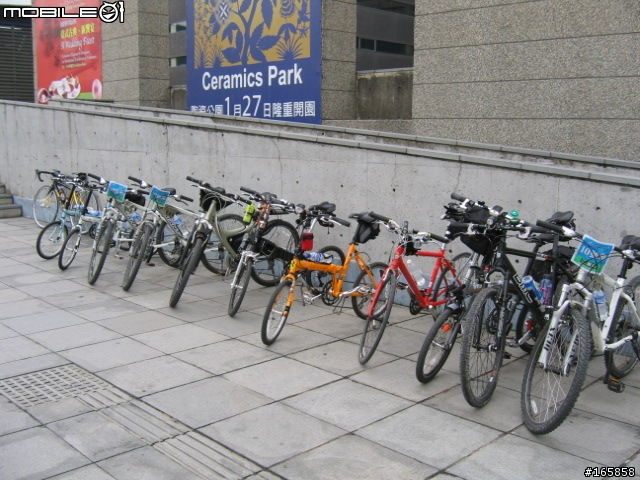In this image, a building with a base made of either granite or cinder blocks features prominently. The structure is slightly slanted to the back of the frame, and it includes a clear glass window displaying two distinct posters. One poster, characterized by its red color, displays slanted writing that is too distant to decipher. The second poster has a blue background adorned with blue leaves inside a gold square, and it reads "Ceramics Park 127." Additional text in another language is present, along with the number "165858" found in the bottom right corner of the photo. The top left corner of the image bears the word "MOBILE" in all caps, accompanied by a small logo depicting a round head with two horns, a white circle with two eyes, and an inverted triangle mouth.

The foreground features a neatly tiled white sidewalk bordered by a stone wall. Approximately 15 bicycles are lined up in front of the building, some propped on their kickstands while others rest against each other. The bicycles come in a variety of colors, including white, black, red, orange, green, yellow, and blue. A drainage grate is visible at the bottom left of the image, indicating an area for water runoff.